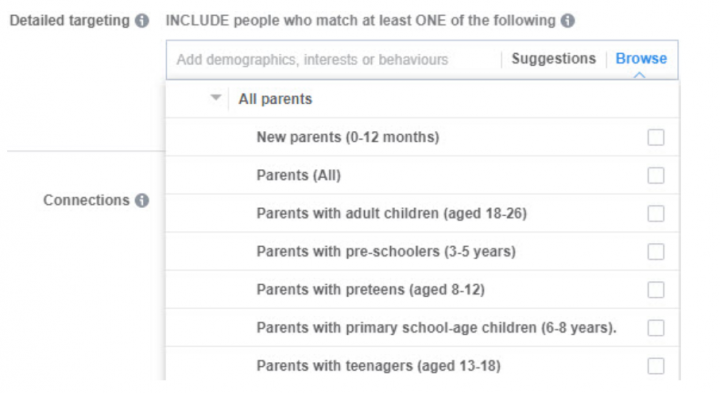This image portrays a simple, white form designed for detailed targeting, likely used for segmentation in a marketing or educational context. The prominent heading reads "Detailed Targeting," followed by a directive to "Include people who match at least one of the following." Most text is in black, with a structured and clean layout.

Beneath this heading, there's an instruction to "Add demographics, interests or behaviors," with "behaviors" spelled with a British English flair, indicating a UK origin. Below this, a "Suggestions" section appears, accompanied by a dark blue "Browse" button with an arrow pointing upward.

The subsequent portion of the form details various categories of parents, including: "All parents," "New parents (0-12 months)," "Parents with adult children," "Parents with preschoolers," "Parents with preteens," "Parents with primary school-age children (6-8)," and "Parents with teenagers (13-18)." Each category has a corresponding checkbox for selection, underscoring the form's comprehensive nature in categorizing different types of parents.